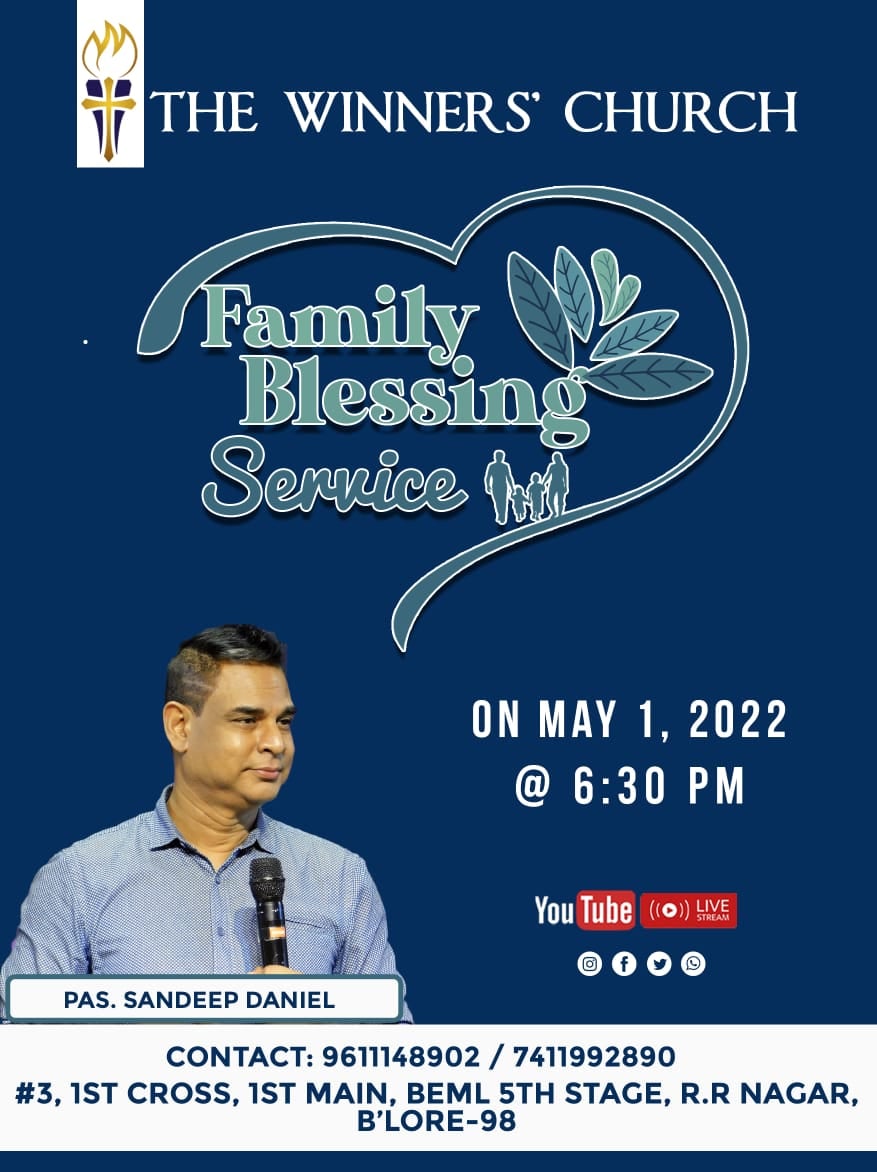The poster is a navy blue advertisement for the Winners Church. At the top, it features a gold-colored cross with a golden flame emerging from it. Below this logo, in white font, the text reads "The Winners Church." Beneath that is the outline of half a heart in green, with the words "Family Blessing Service" inscribed inside. Green leaves extend from the "G" in "Blessing." The heart also contains a small silhouette of a family, consisting of a man and a woman holding hands with two children between them.

In the lower left corner of the poster, there is an image of Pastor Sandy Daniel, who appears to be of Indian descent. He is shown from the chest up, wearing a muted blue button-down collared shirt, with short, closely cropped black hair, and holding a microphone while looking to the right. His name, "Pastor Sandy Daniel," is printed below the picture in a white rectangle.

In the lower right corner, the text "May 1st, 2022 at 6:30 p.m." is displayed in white font. Below this, various social media icons for YouTube, Twitter, Facebook, and Instagram are arranged alongside a telephone icon. Further down, in dark navy text, the contact information is provided: "Contact 961-111-48902 / 741-1992-890." The address reads, "No. 3, First Cross, First Main, BEML, Fifth Stage, R.R. Nagar, BLR-98," with a thick black line beneath this information.